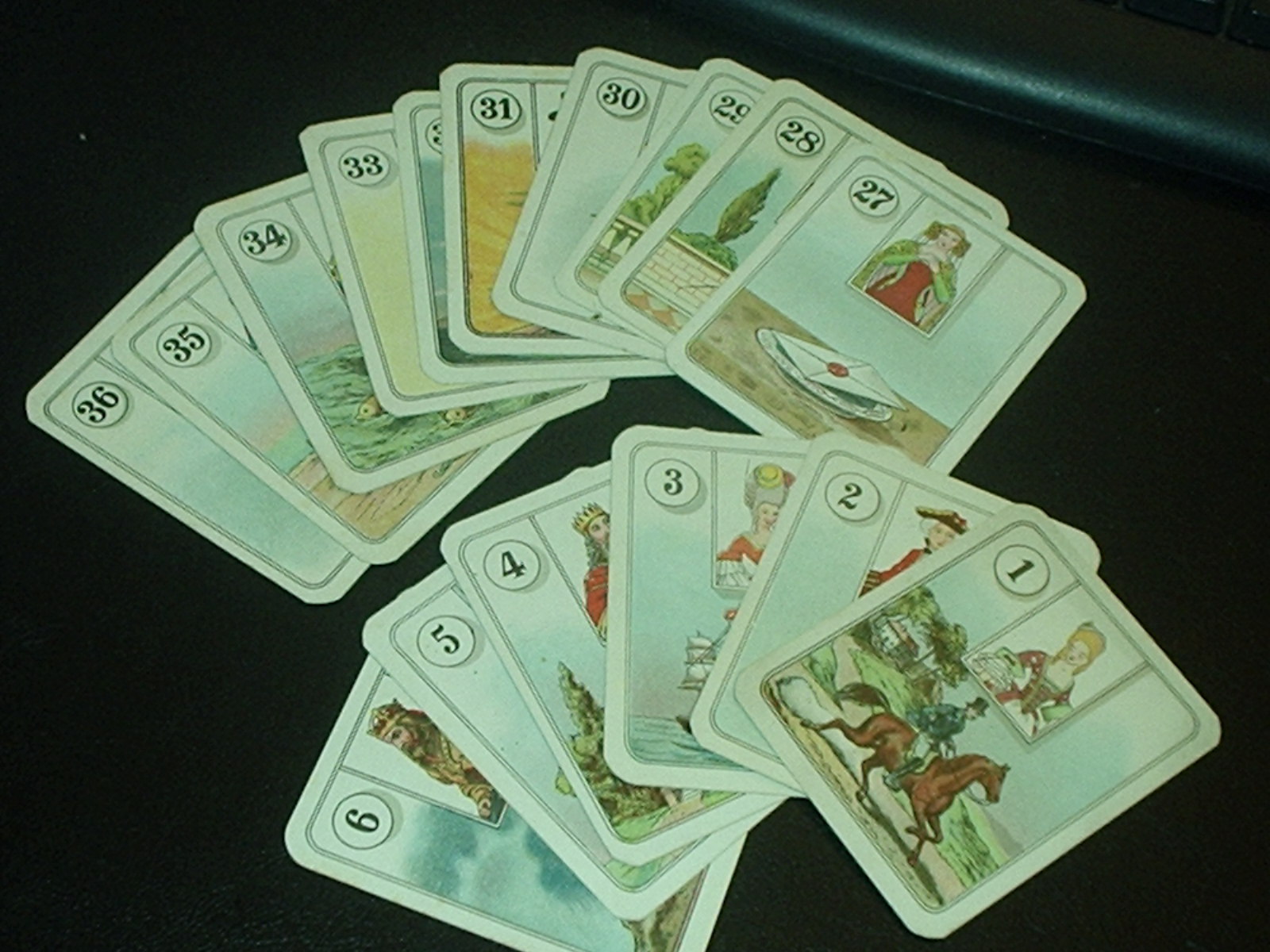The image showcases a collection of scattered cards on a black table, arranged without any discernible order. The cards are divided into two groups: ten cards are spread across the top of the table, while six cards are placed together near the bottom.

The top set of cards are predominantly white and feature various illustrations. The cards are numbered as follows, from left to right: 35, 34, 34, 35, 36, 35, 34, 33, 31, 30, 29, 28, and 27. Card number 31 is adorned with a depiction of sand, while card number 28 shows an image resembling a tree. Card number 27 presents a female figure dressed in a red dress paired with a green cardigan. This scene also includes a table on which sit a white envelope with a red seal and a white plate.

The six cards at the bottom are numbered consecutively from 6 to 1. Card number 6 depicts a cloudy scene with a male figure donning a crown and sporting notable hair. Card number 4 features another male figure wearing a crown and a red coat. Finally, card number 1 portrays a woman in a red dress, accompanied by an illustration of a man riding a brown horse just below.